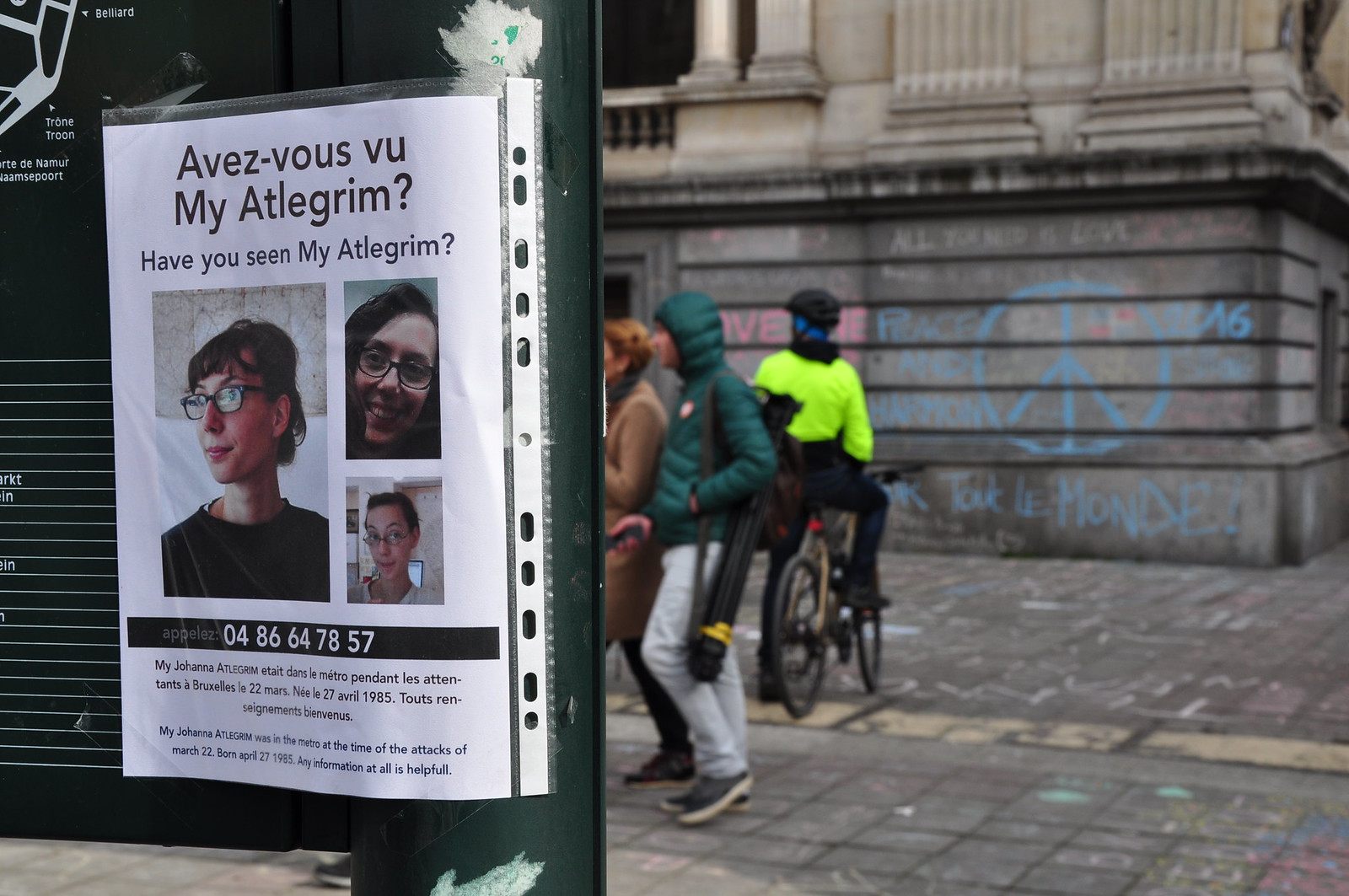The image depicts a lively street scene set against an older gray concrete building adorned with graffiti, including a light blue peace sign and partly legible words. The foreground features a gray brick sidewalk, bustling with people. A person in a neon yellow jacket and black pants rides a bicycle, while another individual in a green hooded jacket and gray sweatpants, with a black item possibly a yoga mat slung over their shoulder, stands nearby. Next to them is a woman with red hair wearing a light brown jacket. To the left, a green lamppost bears a laminated missing person flyer written in French and English, pleading for information on a woman with multiple photos displayed, along with a contact phone number.